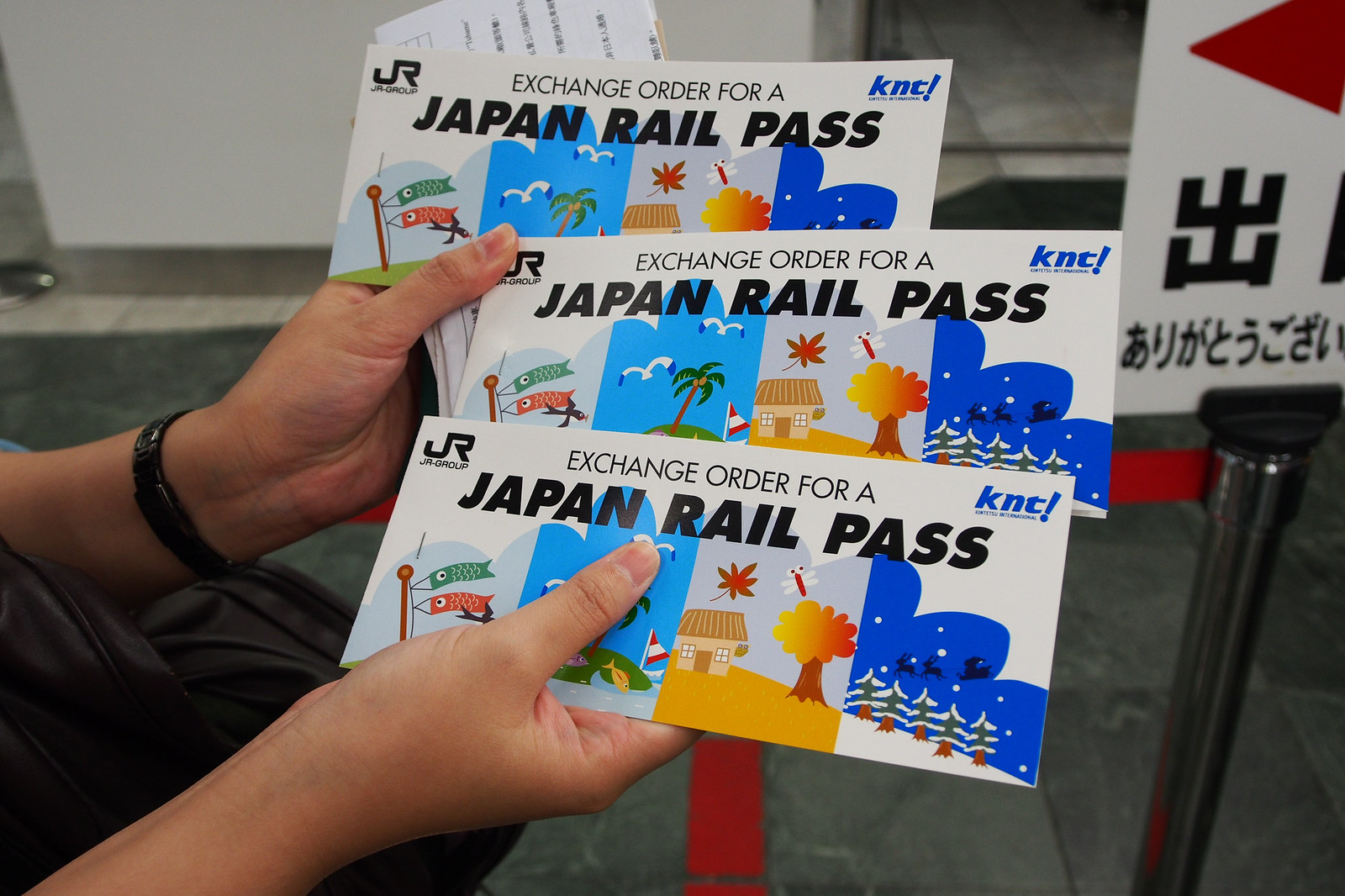In the image, a person—whose gender appears to be female based on the well-manicured nails—is holding three Japan Rail Passes in their left hand. The passes are prominently rectangular with a white background and a colorful design that features hues of blue, light gray, and various other colors. The passes are divided into four sections, each depicting different scenes: a fish on a windsock, seagulls flying over an island, a house surrounded by trees with autumn leaves and a dragonfly, and Santa Claus with reindeer flying over a snowy forest. Each pass also includes the text "Exchange Order for a Japan Rail Pass", the JR Group logo in black at the top left, and the K&T logo in blue with an exclamation point at the top right. The person is wearing a black wristband or watch on one hand. The background features an indistinct sign with Asian characters, set in a drab gray room.